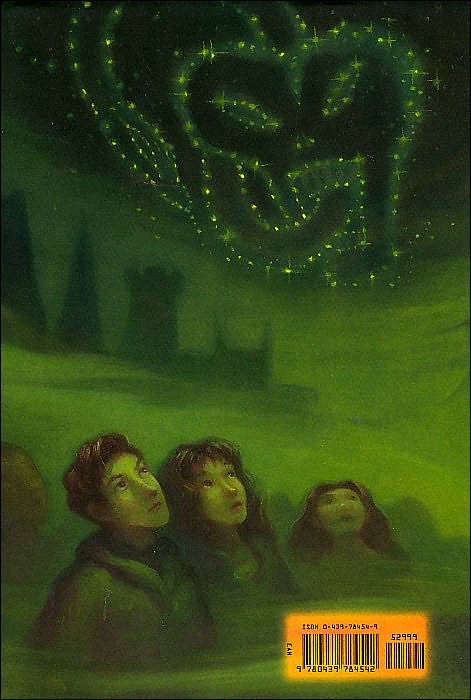This detailed image showcases the back cover of the book "Harry Potter and the Half-Blood Prince." The predominant color theme is shades of green, creating a mystical and eerie atmosphere. In the middle and lower section of the cover, there's a group of characters, including what appears to be Harry Potter with short hair and a green jacket, Hermione Granger with long brown hair, and another young woman with long hair. They are all gazing upwards with expressions of amazement. In the sky above them, twinkling green stars form a sinister visage resembling a skull with a snake emerging from it, an iconic representation of the Dark Mark. Below the stars, there is a silhouette of a mysterious castle on a hill, adding to the magical ambiance. On the bottom right-hand side, there is a yellow rectangle housing two barcodes, the larger one displaying the numbers 4780939784542 and a smaller barcode labeled with the numbers 52999.